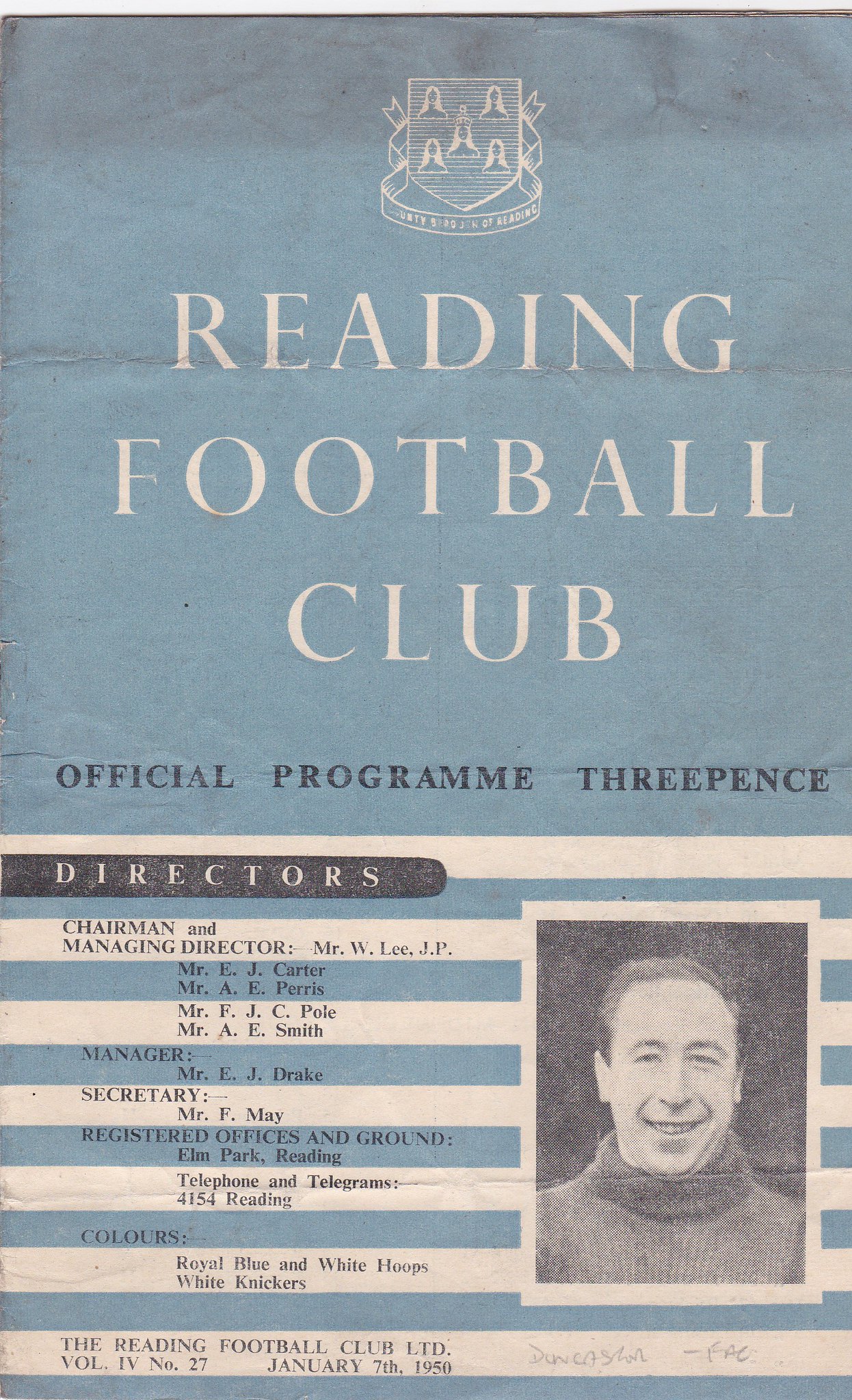The image features a scanned front cover of an old Reading Football Club program set against a light blue background. At the top center, a shield logo with a banner flanked by four R's (two on each side) in white letters prominently displays "Reading Football Club." Directly below, in smaller black text, "Official Program 3 Pence" is visible. Below this, a black banner labeled "Directors" lists several names, including Chairman and Managing Director Mr. W. Lee, along with titles for Manager, Secretary, Registered Offices, and Ground Colors. The lower half of the cover is adorned with alternating blue and white stripes. On the right side, there is a large black-and-white photograph of a smiling man wearing a turtleneck sweater. The bottom line of the cover, in black letters on a white background, reads "The Reading Football Club Limited, Volume 4, Number 27, January 7, 1950."